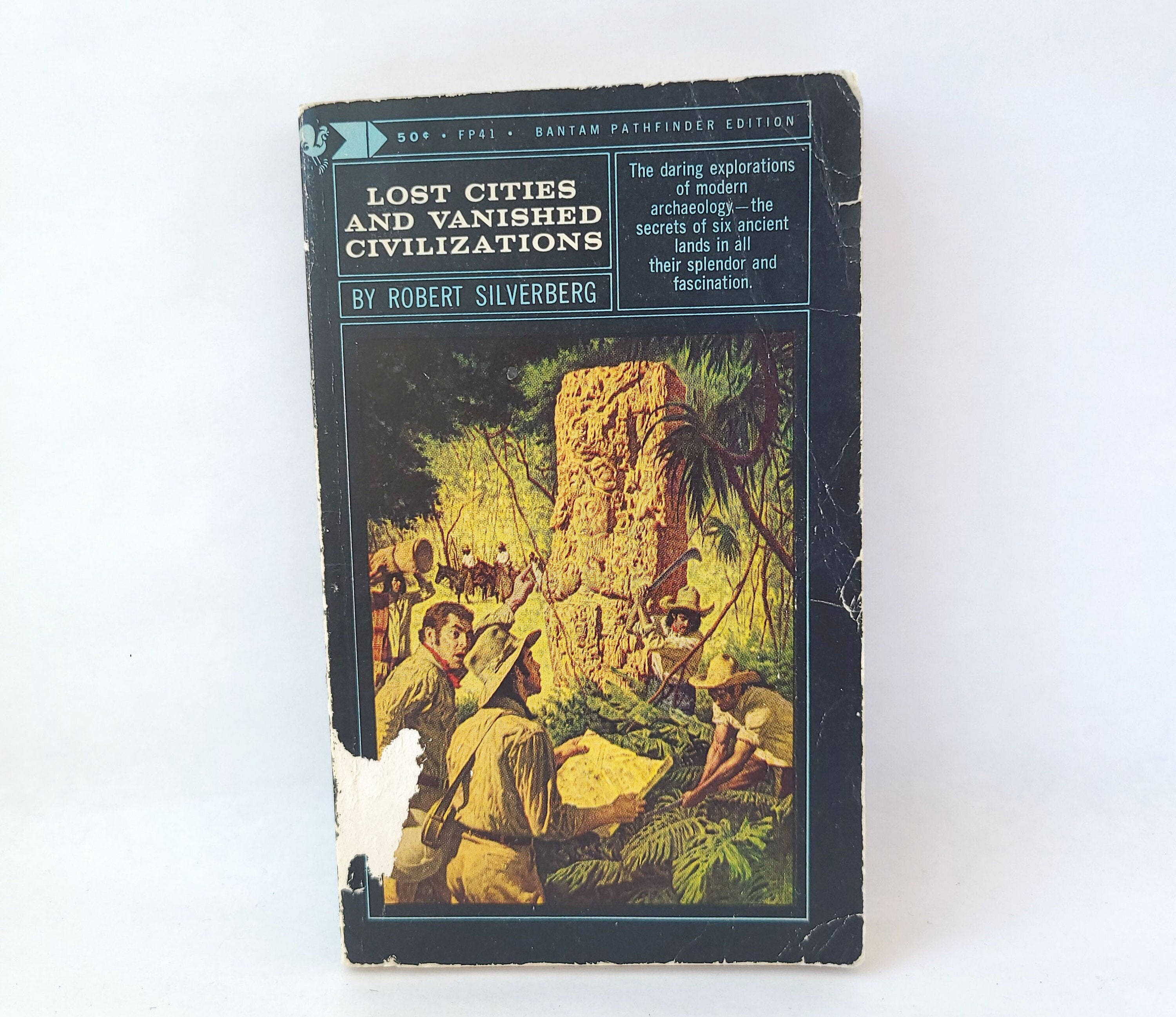The image features the cover of an old paperback book, characterized by its worn and creased appearance. The book is titled "Lost Cities and Vanished Civilizations" by Robert Silverberg, highlighted in white capital letters, with additional text in blue stating "The Daring Explorations of Modern Archaeology, The Secrets of Six Ancient Lands, and All Their Splendor and Fascination." At the top of the cover, it reads "50 Cents FP1 Bantam Pathfinder Edition." The illustration on the cover depicts a lively scene of people in safari outfits, resembling explorers or archaeologists in a dense jungle setting. One man is holding a map, while another is engaging with plants, possibly cutting them down. The vibrant colors of green, blue, yellow, black, and white enrich the scene, giving it a vivid and adventurous vibe akin to an Indiana Jones expedition.